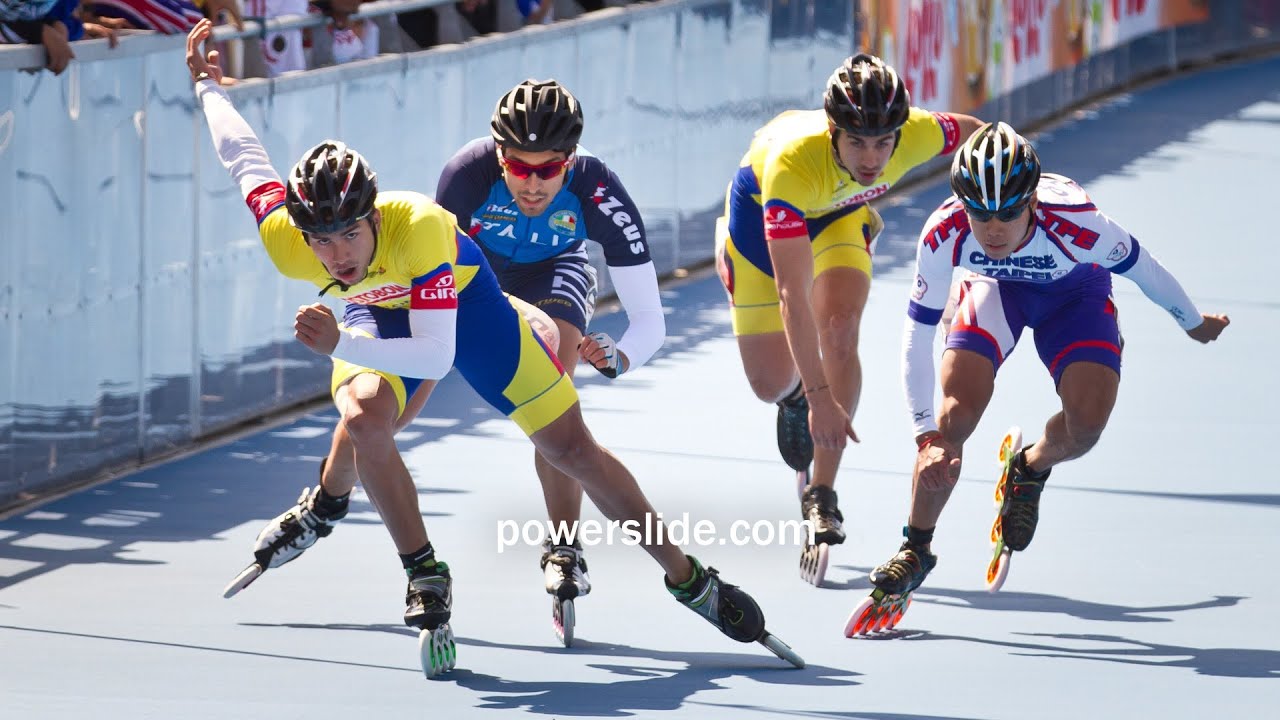This photograph captures a dynamic scene of four men racing in an inline skating competition. The setting is outdoors during the daytime, as evidenced by the shadows cast to the right of the skaters. All four men are dressed in brightly colored, aerodynamic uniforms designed for minimal wind resistance, reminiscent of cycling gear. Each wears a black helmet, similar to those worn by bicyclists. The skaters are on a gray concrete surface, moving past a white rail that lines the outer edge of their path. 

From left to right, the first skater, swinging his arms, is clad in a multicolored outfit featuring yellow, blue, white, and red. The second man wears a blue, black, and white ensemble, closely trailing the first. The third skater, similar in appearance to the first, also sports a yellow, blue, red, and white uniform. Finally, the fourth individual on the far right is dressed in red, white, and blue. All four skaters appear to be in full stride, leaning forward with a sense of urgency and determination. In the background, the words "powerslide.com" are prominently visible, reinforcing the competitive nature of their activity.